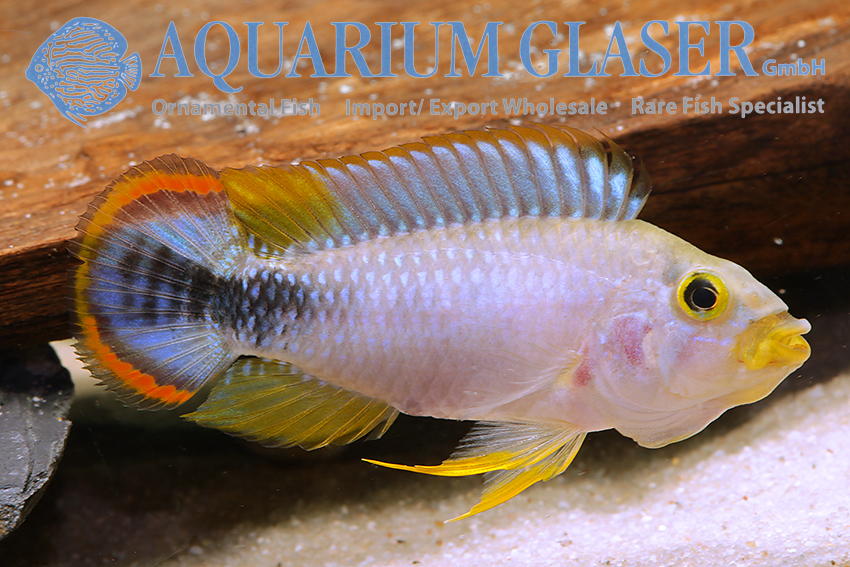The image, titled "Echorium Glaza GMBH Allimental Fish Import/Export Wholesale Rare Fish Specialists," prominently features an exquisite white fish facing left. This striking aquatic creature has vivid blue eyes encircled by a black ring and a distinctive yellow mouth. The dorsal fin is predominantly silvery white, transitioning to yellow toward the tail. Its ventral fin displays a bright yellow hue, while the pectoral fins are a combination of white and yellow. The tail fin showcases a captivating array of colors, with an orange semicircle near the end, and a complex pattern of white, black, and silver coloring.

The scene is set against a backdrop of a brown wooden log and an aquarium environment with sand at the bottom and noticeable air bubbles. Above the fish, the company’s logo—a blue fish—is featured along with the name "Aquarium Glacier GMBH." The text beside the logo reads "Ornamental Fish, Import/Export Wholesale, and Rare Fish Specialists," suggesting an advertisement for the company's aquatic services.